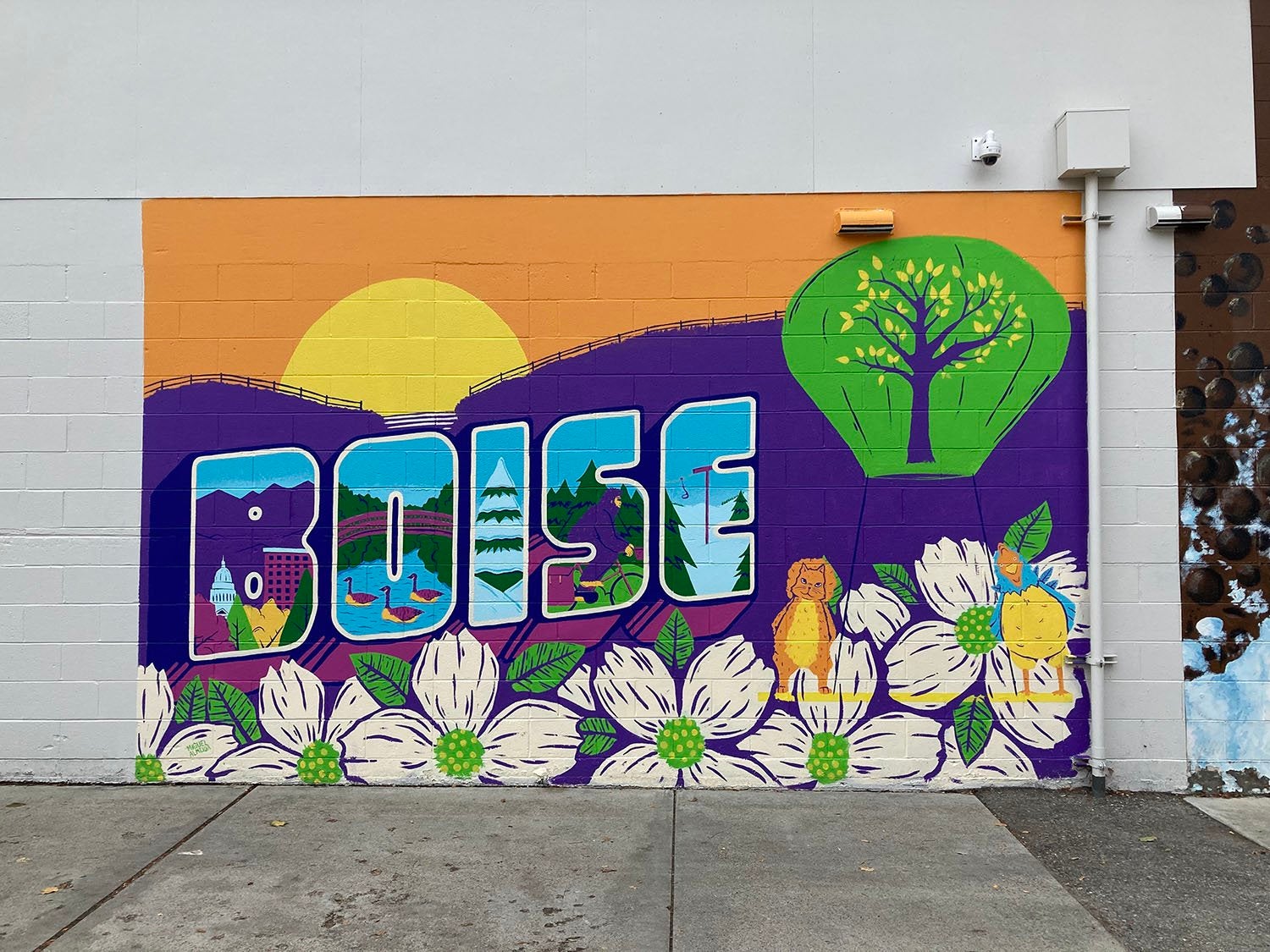The image showcases a vibrant and detailed wall mural painted on the side of a brick building, transforming what would otherwise be an unremarkable edifice into a captivating artwork. The mural prominently features the word "Boise" in large, bubble-like, bold letters that span diagonally from the left towards the center right of the wall. Each letter in "Boise" encapsulates elements intrinsic to Boise, Idaho’s natural and cultural scenery. For instance, the 'B' is filled with images of city buildings, the 'O' contains geese, and other letters depict snowy trees, a body of water, a skiing scene, and a tractor, adding layers of local significance.

The backdrop of the mural depicts a nature scene with a dam, a stylized tree, and a vibrant sky transitioning into what appears to be either a sunrise or sunset, painted in hues of yellow and orange. The bottom part of the mural features large, white flowers with green centers, adding to the mural’s enchanting aesthetic. Amidst this flora, a squirrel or rodent and a chicken-like animal are seen standing together, contributing to the lively and whimsical atmosphere.

A striking feature of the mural is its simplistic graffiti style, characterized by bold, solid colors and clean outlines. The area surrounding the mural is painted in a light grey, subtly directing focus to the colorful center. Above the mural is a security camera, a modern observer of the mural and its surroundings. The scene is captured on an overcast day, where the light is diffused, enhancing the mural's vivid colors and details. The overall composition is nicely centered, underscoring the mural's role in beautifying the street and celebrating Boise’s unique charm and natural beauty.